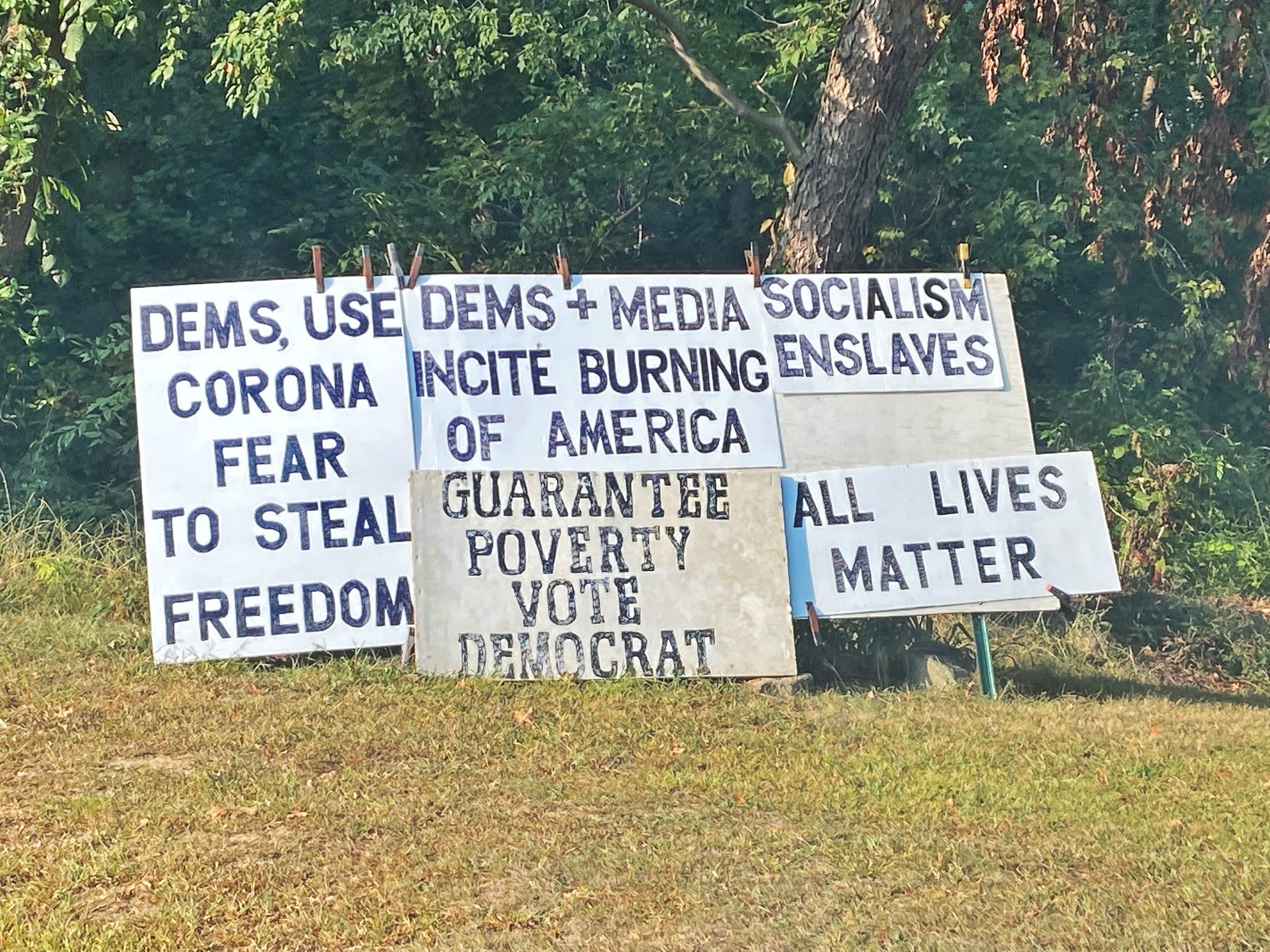In the image, three white poster board signs are prominently displayed, each featuring bold black block lettering. The signs are pinned to a backdrop and positioned on slightly brown grass, in front of a cluster of trees adorned with green leaves. 

The first sign, on the left, reads: "Dems use Corona fear to steal freedom." The center sign declares: "Dems + media incite burning of America, guarantee poverty, vote Democrat." The third sign on the right states: "Socialism enslaves," followed by the phrase, "All lives matter."

The scene captures a heavily opinionated political message amidst a natural setting, where the green foliage of the trees contrasts with the brownish tinge of the grass, adding a sense of grounded realism to the stark and provocative statements on the signs.